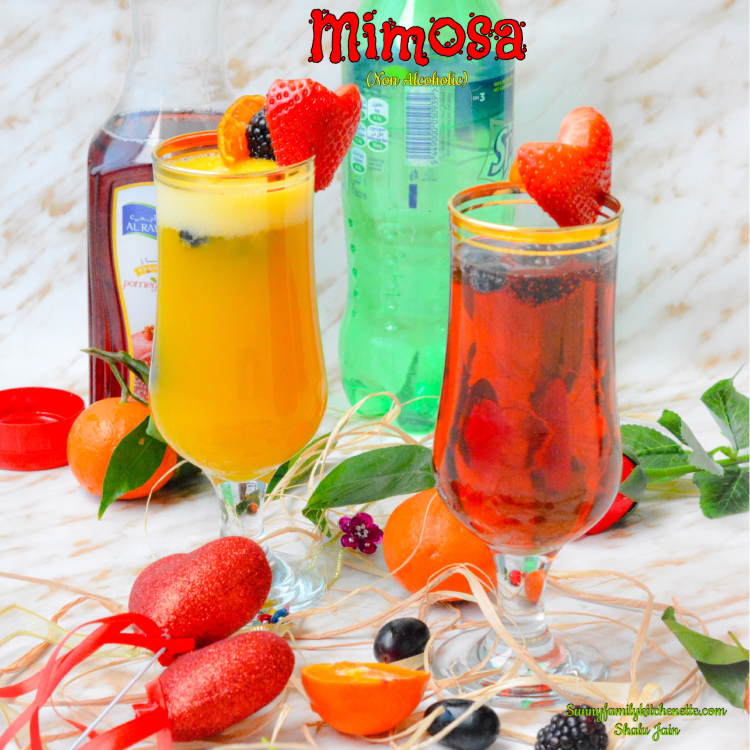The image is a professional photograph of two elegantly presented drinks set against a white marble backdrop with beige veining. Both drinks are in clear glasses with gold rims, each fashioned with an upside-down bell-shaped body, a glass stem, and a base. The glass on the left contains a bright yellow, foamy liquid, garnished with a heart-shaped strawberry slice, a blackberry, and a small kumquat wedge. The glass on the right is filled with a clear red liquid, with blackberries floating inside and topped with a similar heart-shaped strawberry slice. Surrounding the drinks are vibrant ingredients including half an orange, additional oranges, more blackberries and strawberries, and some green leaves, adding to the colorful presentation. Decorative heart-shaped ornaments with red ribbons are interspersed among the ingredients. Behind the glasses are two bottles: a red bottle labeled "pomegranate" on the left, and a green bottle of Sprite on the right with "Mimosa" written on it. Additional details include a barely readable URL "SunnyFamilyKitchenette.com" in green cursive text at the bottom right of the image.